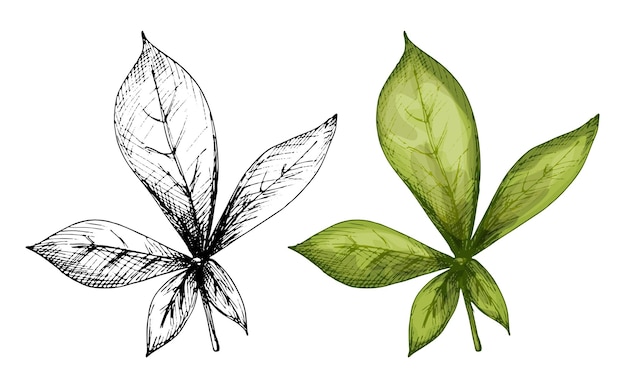The image consists of two drawings of the same five-leaf plant, one black-and-white and one colored. On the left, the black-and-white sketch shows a detailed pencil or ink drawing, depicting a large central leaf at the top, flanked by two medium-sized leaves on either side, and two smaller leaves at the bottom. The etching lines are intricate, illustrating the veins and texture of each leaf. On the right, the same leaf arrangement has been filled in with varying shades of olive green, showcasing a cohesive yet subtly nuanced color scheme. The line work in the colored image is still visible but less pronounced, slightly muted by the green tones. The leaves exhibit a slight curl, almost resembling fresh basil, with lighter green highlights indicating where the light hits and darker green edges suggesting shadows, giving the leaves a mildly three-dimensional appearance. The background is completely white, providing a stark contrast that highlights the detailed artwork.